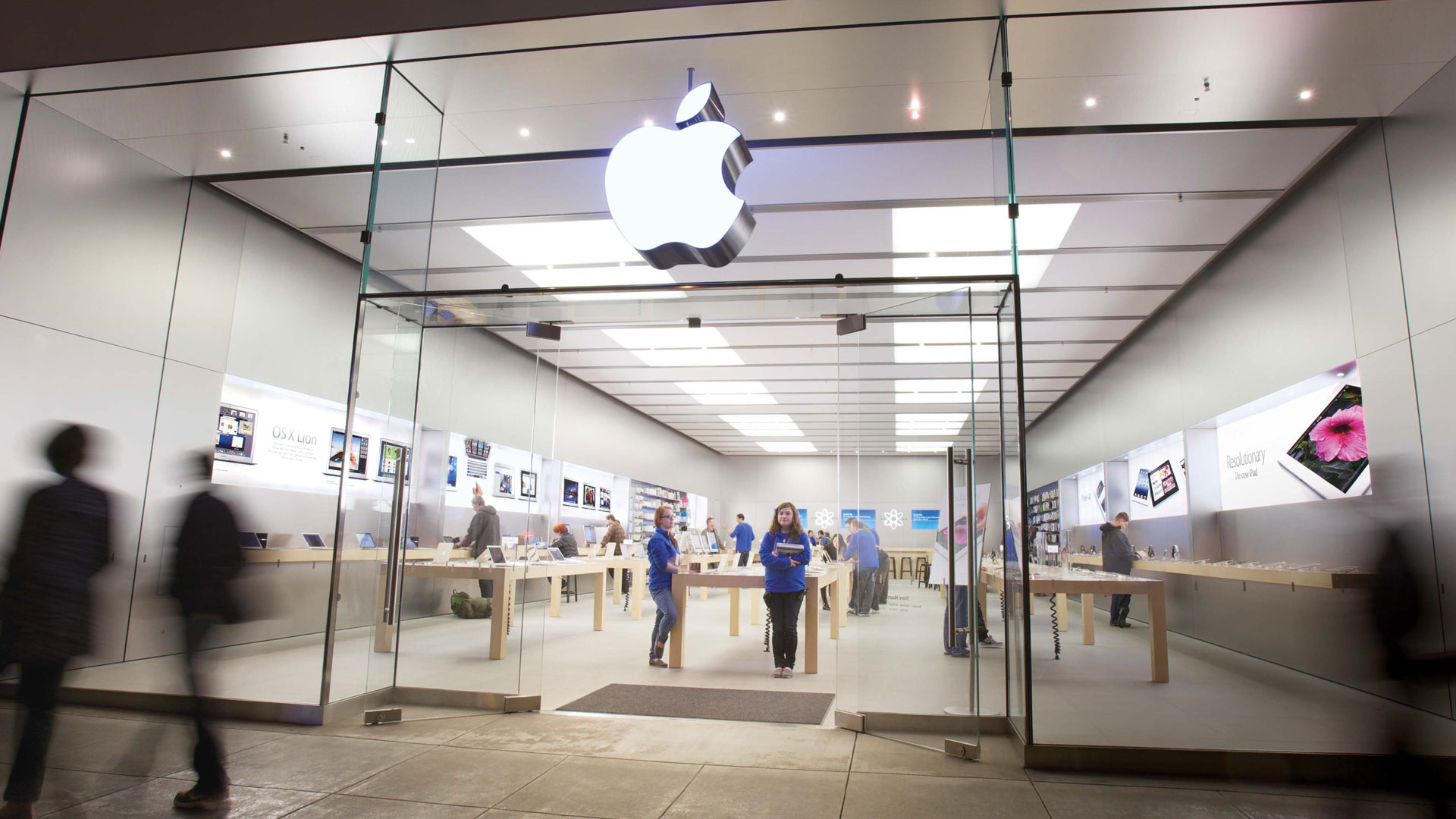A nighttime photograph showcases an Apple Store, likely featured in a magazine or Apple advertisement due to its stylized presentation. The edges of the image are enveloped in darkness, indicating the late hour and the absence of natural light. At the heart of the composition, the Apple Store stands brilliantly illuminated, bustling with activity both inside and out.

Centrally framed, the storefront displays large glass doors and expansive windows, providing a clear view of the interior. Above the entrance, the iconic white Apple logo boldly signals the brand. Inside, blue-clad employees, identifiable by their uniform shirts paired with either black pants or jeans, assist customers amidst the bright, inviting space.

The store's interior features neatly arranged brown tables, each showcasing a variety of Apple products, including iPhones, iMacs, and various accessories, allowing customers to interact with and examine the latest technology. The store's left and right walls are adorned with large screens, likely displaying advertisements or connected to iMacs or iPads for interactive demos. The pristine white floor enhances the store's clean, modern aesthetic.

In contrast, the bottom left of the image captures the blurred silhouettes of passersby on the street, emphasizing the store as the focal point. This well-composed, vibrant vignette effectively highlights Apple's retail experience, suitable for an advertisement on the company's website or other promotional material.